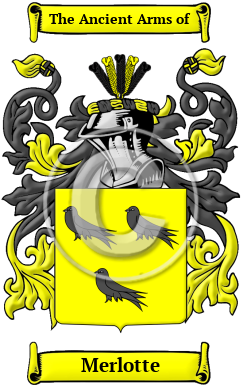The image depicts a detailed emblem design. At the top of the image, there is a yellow banner with black text that reads "The Ancient Arms of." A similar banner is at the bottom, also in black text, reading "Merlot." 

Central to the emblem is a figure facing left, wearing silver armor on his head. Gray strings adorned with leaves extend from the figure; the leaves are gray but turn yellow at the ends. In the center of the design is a yellow, square shield featuring three gray birds, arranged with two at the top and one at the bottom, all facing left. The emblem also includes a gray circle with a transparent "C" in the middle, flanked by the strings extending from the armored figure. This composition presents a blend of medieval and natural elements in its design.